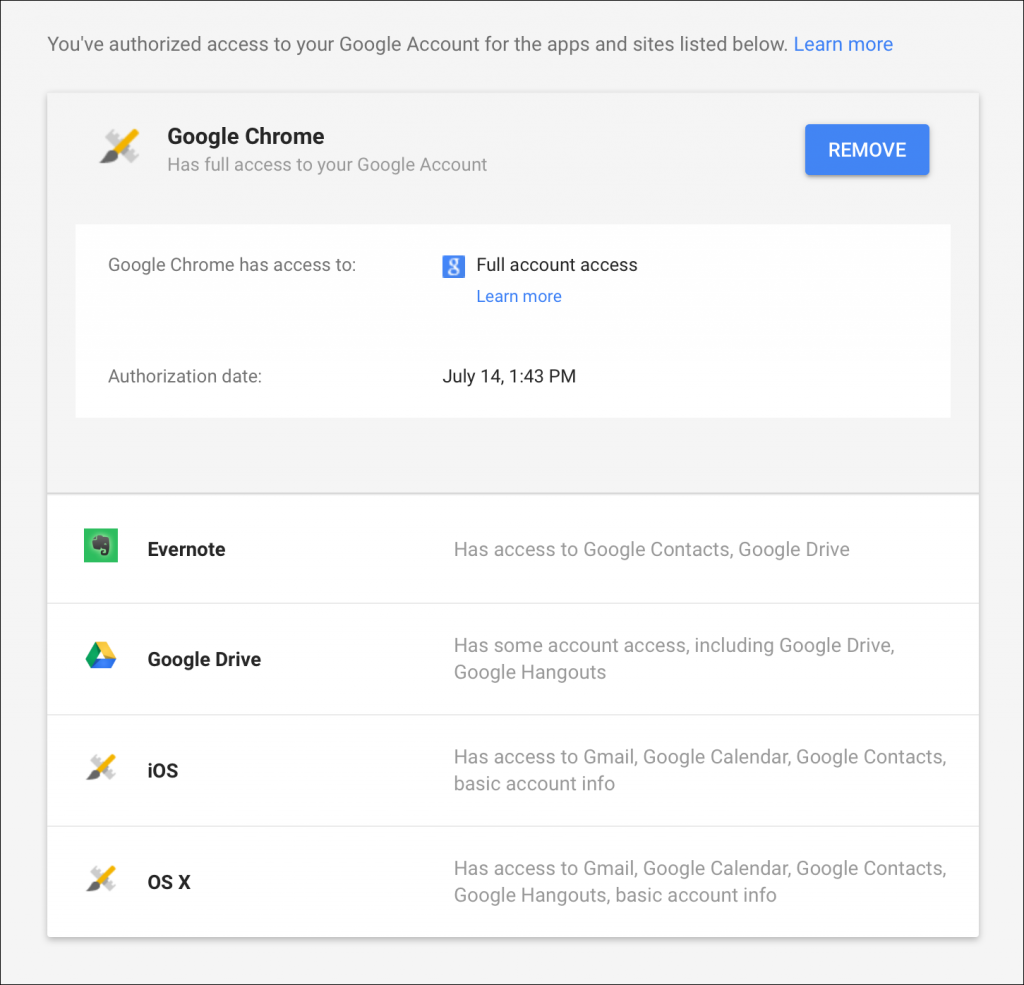This screenshot from Google Chrome's settings page features a light grey background. At the top, in dark grey text, a message reads, "You've authorised access to your Google account for the apps and sites listed below." A "Learn more" link, colored blue, follows immediately after.

Below the message, a crossed paintbrush and ruler icon symbolizes Google Chrome, next to which "Google Chrome" is written. Underneath it, a description notes that Google Chrome has full access to your Google account. To the right of this information, a blue tab labeled "Remove" in white text allows you to revoke access.

Further down, detailed information about various apps with access to your Google account is listed:

1. **Evernote**: This app has a green icon featuring a black elephant and has access to Google Contacts and Google Drive.
2. **Google Drive**: This service has some account access, specifically including Google Drive and Google Hangouts.
3. **iOS**: This indicates access to Gmail, Google Calendar, Google Contacts, and basic account info.
4. **OSX**: This shows access to Gmail, Google Calendar, Google Contacts, Google Hangouts, and basic account info.

Additionally, the authorisation date for Google Chrome's full account access is specified as July 14th at 1:43 PM.